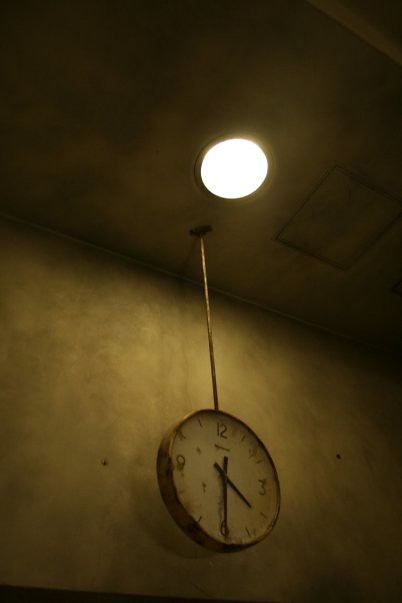In the dimly lit, grimy interior of an old building, a well-worn, heavily rusted clock hangs from the ceiling by a long, cylindrical metal rod. The clock, with its aged and weathered face, only bears the numbers 12, 3, 6, and 9, while the hours in between are marked by simple lines. The clock's white background is stained and faded, and its black hands indicate the time is precisely 4:30. The metal rod is mounted into a circular ceiling bracket, which shows signs of significant rust. The wall behind the clock is textured and dirty, bathed in a dingy yellow and brown hue that adds to the overall eerie atmosphere of the room. Above the clock, a singular cylindrical white light struggles to illuminate the space, casting faint, inconsistent light. To the right of this light, an outline of a square, likely a vent or trap door, is barely visible. The entire scene is enveloped in a sense of decay and neglect, amplifying the room's creepy ambiance.